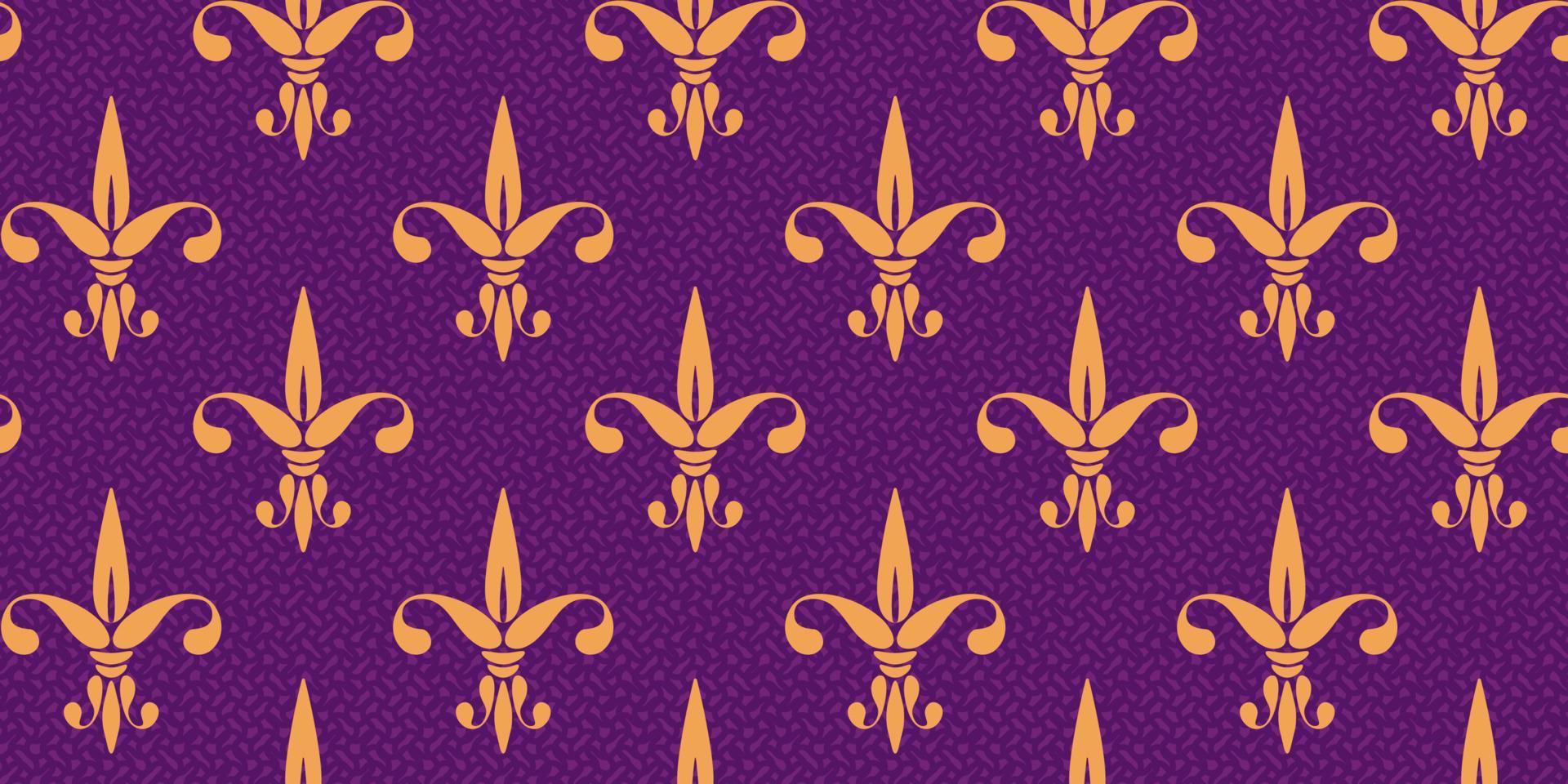The image features a dark purple background sprinkled with very light purple dots, creating a starry effect. Over this backdrop, an array of meticulously designed gold fleur-de-lis symbols is displayed in a repeated pattern, reminiscent of the New Orleans Saints logo. Each fleur-de-lis is elaborately detailed, with a central elongated triangular petal that shoots up, flanked by two curved leaves emanating from the base and bending gracefully back towards the center. The design also includes two circular elements that appear to bind the structure together, as well as additional smaller leaves curving downward and then arching upwards. These gold icons are uniformly distributed across the background in rows, each fleur-de-lis having ample space around it to stand out against the striking purple canvas. The overall effect is both regal and harmonious, blending the historic French symbol with a modern pattern.